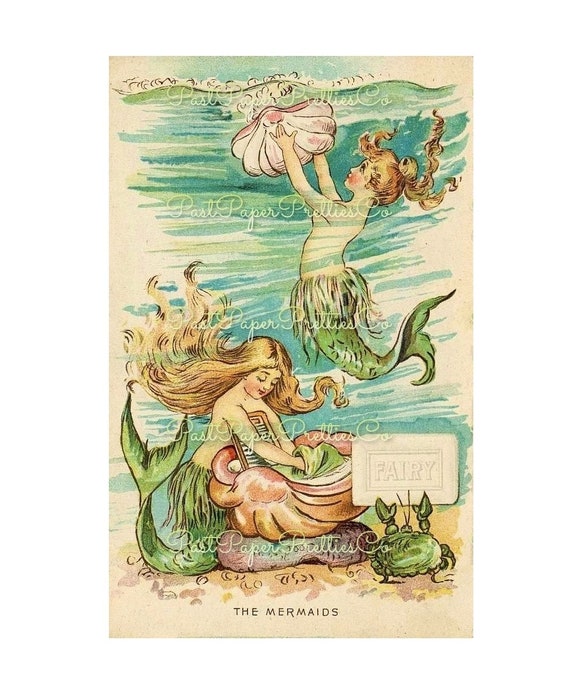This vintage-looking poster, likely a digital recreation or an old advertisement, features an illustration of two angelic, doll-like mermaids. The ivory-colored background and watercolor style contribute to its nostalgic, antique charm. The mermaids, with their long, wavy, light blonde hair and green tails, embody an old-fashioned aesthetic rarely seen today. Wisps of blue and green watercolors suggest the ocean's gentle currents from top to bottom, creating a serene underwater scene.

At the bottom of the poster, a mermaid with no top, resembling a little girl, washes clothes in a giant pink seashell on the sandy ocean floor. Beside her is a green crab holding a bar of soap labeled "Fairy." Above her, another mermaid floats gracefully, holding a pink seashell as if she's lifting it above the ocean. This second mermaid, positioned more towards the top right, also has blonde hair, which appears slightly braided, and a green tail. Both mermaids and the sea creatures are surrounded by a repeating watermark that reads "Past Paper Pretties Co." in a faint, cross-stitched pattern from top to bottom, adding to the illustration's vintage authenticity.